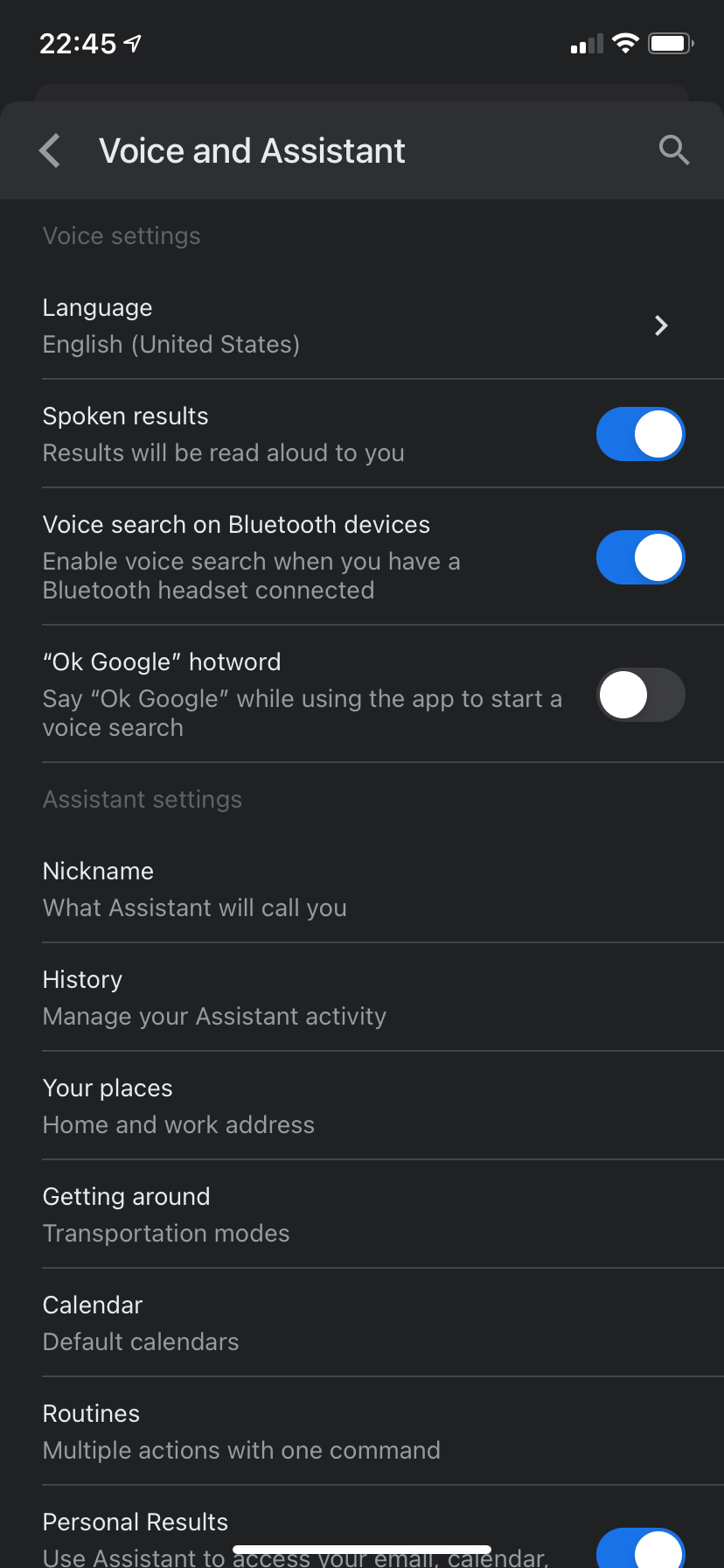The image is a screenshot from a smartphone, displayed in a vertical orientation with a predominantly black background. At the top of the screenshot, the time is shown as 22:45. To the right of the time, the phone's battery icon indicates a full charge, and the volume icon shows that the volume is set to the maximum level. The Wi-Fi signal strength icon reveals a relatively weak connection, with only two out of the possible four bars filled.

Moving further down, the screenshot focuses on a settings section labeled "Voice and Assistance." Within this section, several options are visible:

1. **Spoken Results**: This feature is turned on, allowing the phone to provide audible responses to queries.
2. **Voice Search on Bluetooth Devices**: This option is also activated, enabling voice search capabilities over connected Bluetooth devices.
3. **“OK Google” Hotword**: This feature is disabled, meaning the phone will not respond to the "OK Google" activation phrase.
4. **Personal Results**: This setting, which allows the assistant to access personal information such as the user's calendar, is turned on.

Each of these options is illustrated by icons and toggle switches that clearly indicate their current status, providing a comprehensive view of the user's voice and assistance settings.